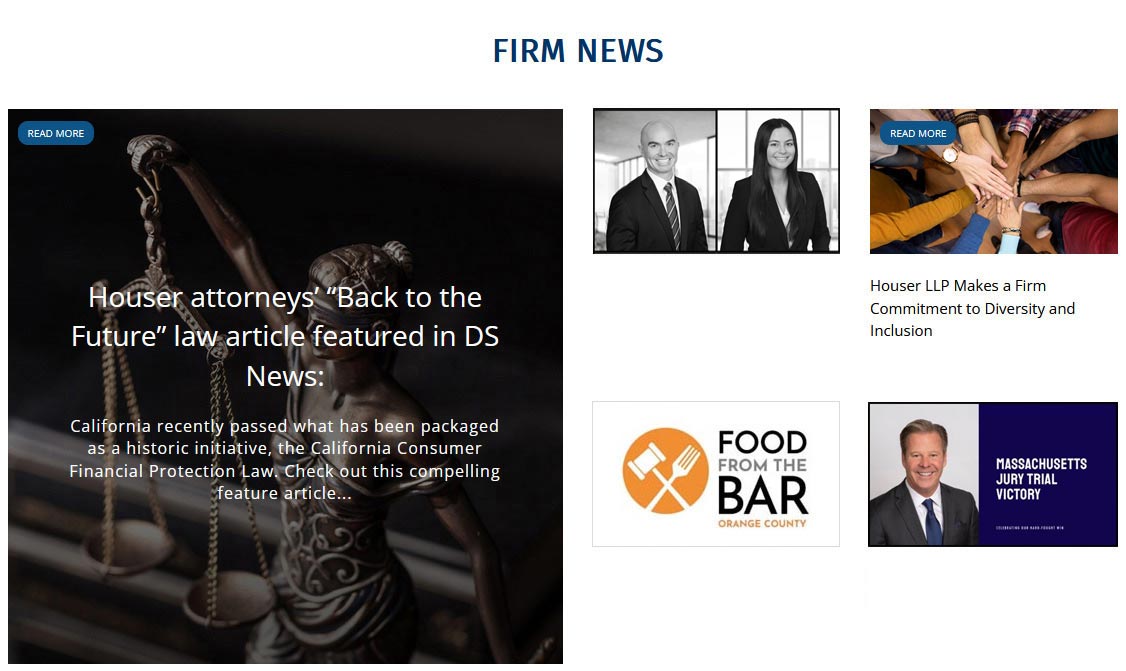This image showcases a firm’s newsletter page, marked by a "Firm News" header in navy blue font against a white background. Dominating the left side is a large square image with a black backdrop, featuring a bronze statue of Lady Justice wearing a blindfold and holding scales. The image includes a blue button labeled "Read More" and white text that reads: "Hauser Attorneys: Back to the Future Law Article Featured in DS News." The accompanying text highlights a historic initiative, noting that California recently passed the California Consumer Financial Protection Law.

To the right of this, a city skyline image is displayed with bold white text announcing a "Legal Issues and Regulatory Compliance Conference." Below this skyline image is another section on a white background, featuring an orange square with a hammer and fork icon, accompanied by the text "Food from the Bar Orange County." 

Additionally, there is an image of a group of people placing their hands together in a collective gesture, captioned "Hauser LLP Makes a Firm Commitment to Diversity and Inclusion." The final image has text reading "Legal Issues and Regulatory Compliance Conference California MBA," reinforcing the focus on legal and regulatory topics. 

Surrounding these central images, a variety of headlines and advertisements are scattered across the page, creating an informative and visually engaging layout.